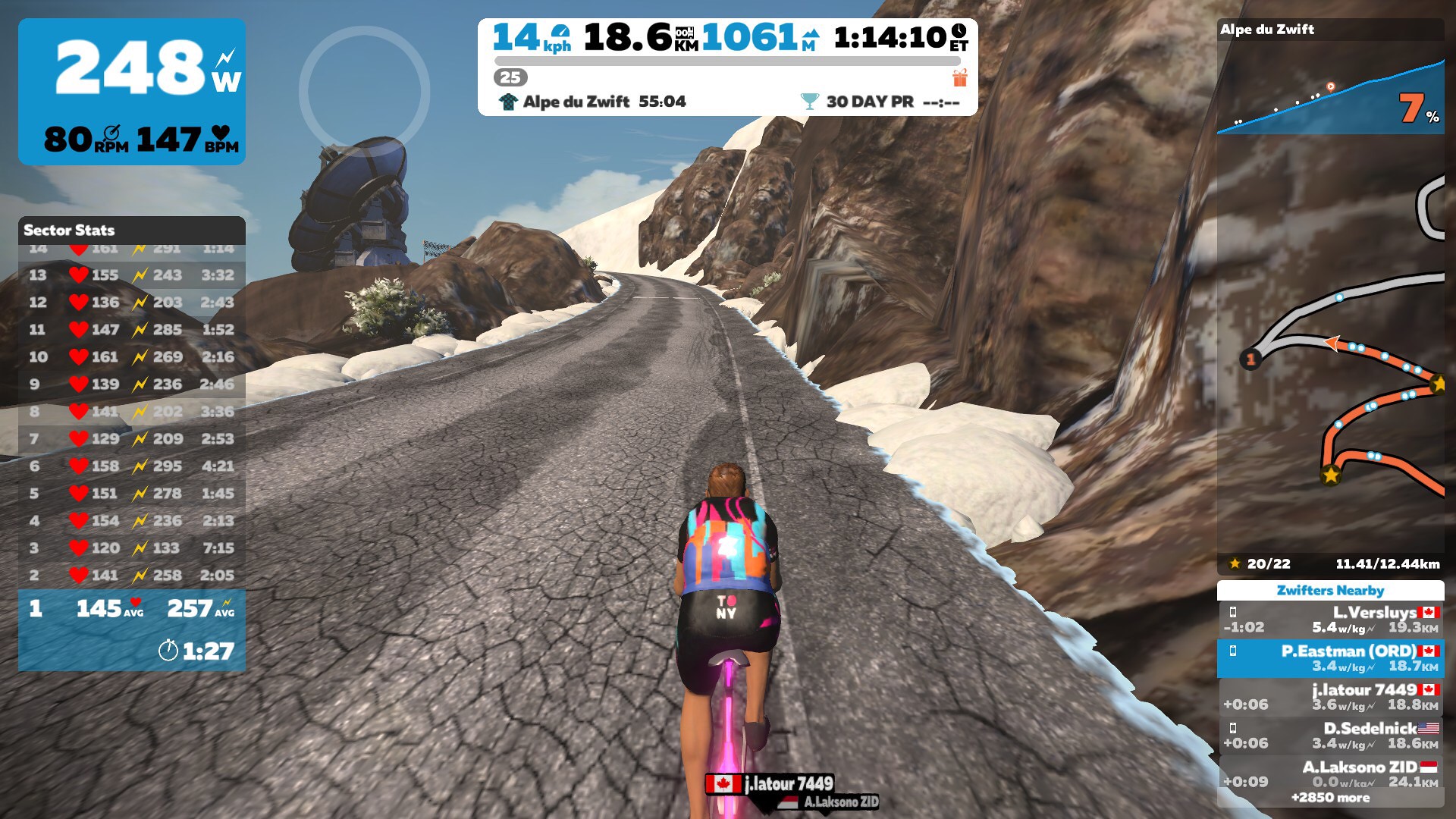The screenshot appears to be from a virtual cycling app, likely Swift Cycling or a similar platform. It showcases a rider's avatar cycling up a cracked gravel road on a pink bike, with the phrase "To New York" printed on their shorts. The scene is set on a mountain road, bordered by patches of snow. On the top left corner, the screen displays various performance metrics: "248 Watts," "80 RPM," and "147 BPM," followed by a leaderboard. Centrally, the display indicates speed, distance, elevation, and elapsed time: "14 kph," "18.6 km," "1061 m," and "1 hour, 14 minutes and 10 seconds ET." A mini-map runs along the right side, from top to roughly the bottom middle, providing further context to the rider's journey.